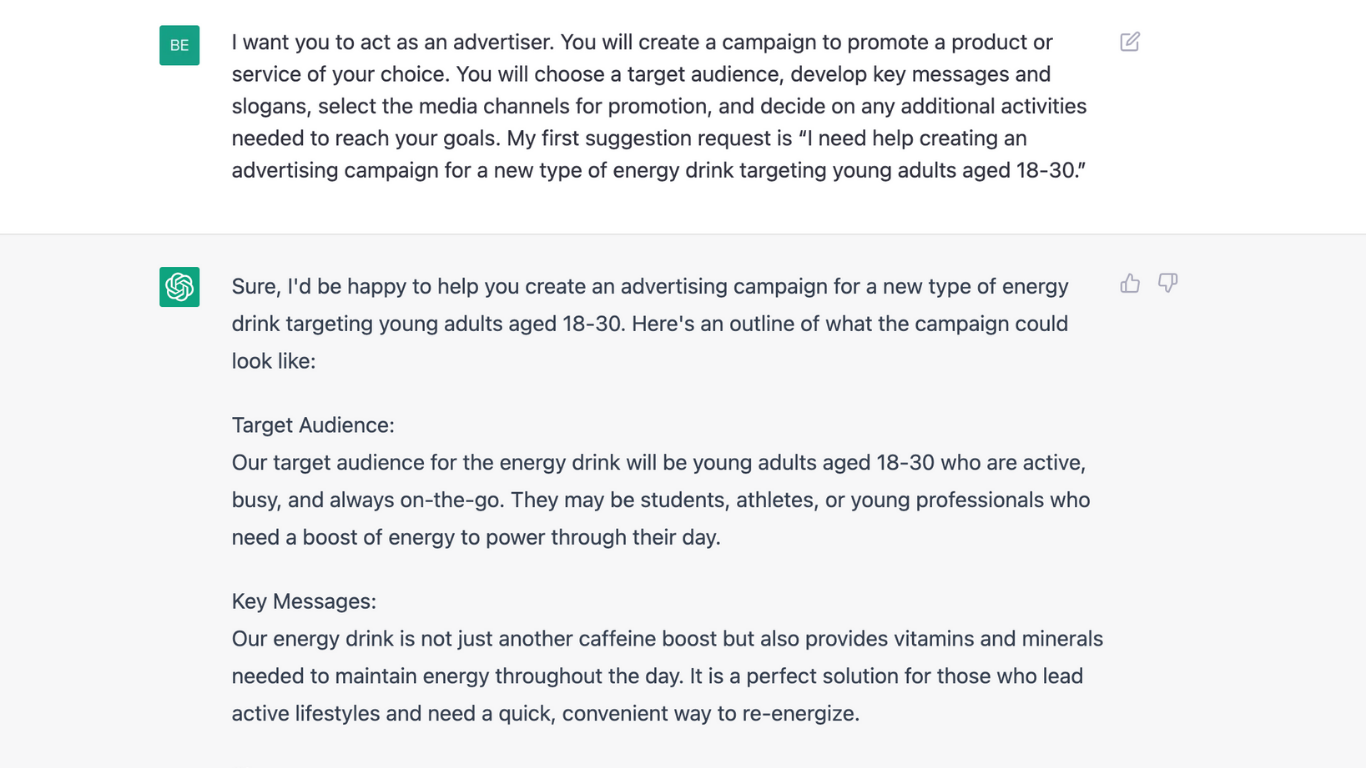The image showcases a webpage featuring an interaction with a chatbot. The top section of the webpage displays a green square with the initials "BE" prominently highlighted. Below it, there is a text box containing a user prompt that reads: 

"I want you to act as an advertiser. You will create a campaign to promote a product or service of your choice. You will choose a target audience, develop key messages and slogans, select the media channels for promotion, and decide on any additional activities needed to reach your goals. My first suggestion request is, I need help creating an advertising campaign for a new type of energy drink targeting young adults aged 18-30."

Following this prompt, there is a chatbot reply:

"Sure, I'd be happy to help you create an advertising campaign for a new type of energy drink targeting young adults aged 18-30. Here is an outline of what the campaign could look like:

**Target Audience:** Our target audience for the energy drink will be young adults aged 18-30 who are active, busy, and always on the go. They may be students, athletes, or young professionals who need a boost of energy to power through their day.

**Key Messages:** Our energy drink is not just another caffeine boost, but also provides vitamins and minerals needed to maintain energy throughout the day. It is a perfect solution for those who lead active lifestyles and need a quick, convenient way to re-energize."

The page background is a blend of grey and white tones, and the text is rendered in black for clear readability. Additionally, there are thumbs up and thumbs down icons present, presumably to allow users to rate the chatbot's response.